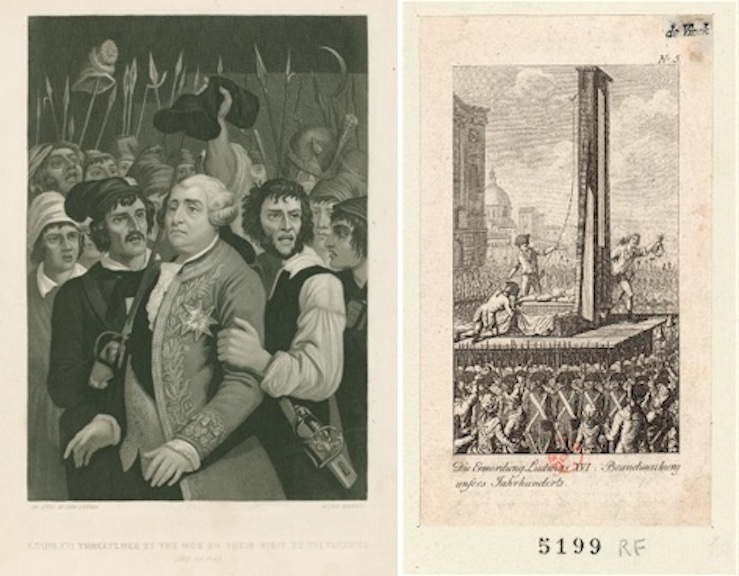This historical photograph captures an open pamphlet displaying two detailed, black-and-white illustrations from the French Revolution, set against a sepia-toned background. The left page portrays a somber scene of a stoic King Louis XVI, clad in a long red coat adorned with a star and wearing a white curly wig, being forcefully led away by a furious mob brandishing spears, pitchforks, and scythes. This group of commoners is clearly angry, embodying the revolutionary fervor of the period. On the right page, the illustration depicts the grim aftermath: a guillotine starkly positioned, with an execution underway and a crowd gathered to witness the event. Soldiers form a protective phalanx around the guillotine platform, adding to the tense atmosphere. This image is punctuated by the presence of attendants preparing the execution apparatus amidst what is presumably a Parisian background with cloudy skies. The illustration bears a reference number "5199" and the hand-printed letters "RF," suggesting historical authenticity. The pamphlet, characterized by its vintage and possibly mid-18th century etching style, lends a haunting glimpse into one of history's most tumultuous periods.